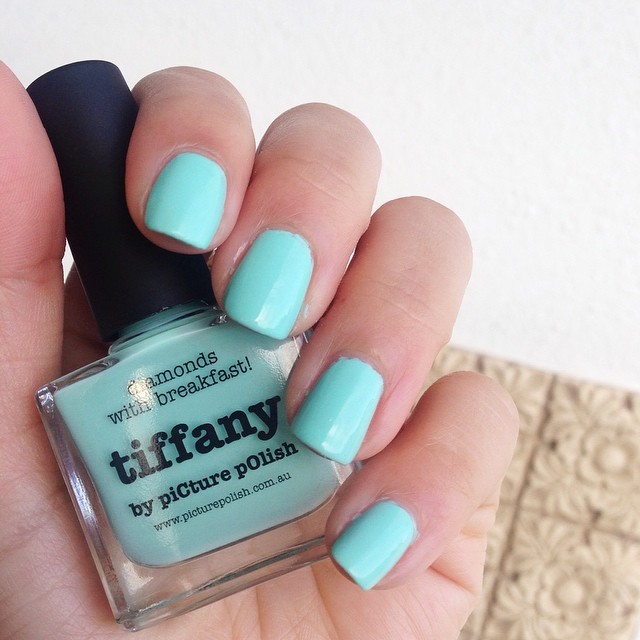This close-up square photograph showcases a hand clutching a bottle of nail polish. The nails, painted in a very light teal, almost akin to a robin's egg blue, perfectly match the polish in the bottle they hold. The thumb is not visible, but the other four nails are prominently displayed, showing off the smooth and even application of the polish. The clear glass bottle, still full, features a bold black cylindrical cap. Black text on the bottle reads, "Diamonds with Breakfast Tiffany" by Picture Polish, with "Tiffany" standing out due to its larger and bolder font. The background presents a distinctive half wall: the upper portion is a clean white, while the lower part is adorned with ornate, square, clay tiles, each designed with a central flower motif surrounded by leaves. This elegant setting provides a delightful contrast to the vibrant, serene color of the nail polish, enhancing the overall aesthetic of the photograph.